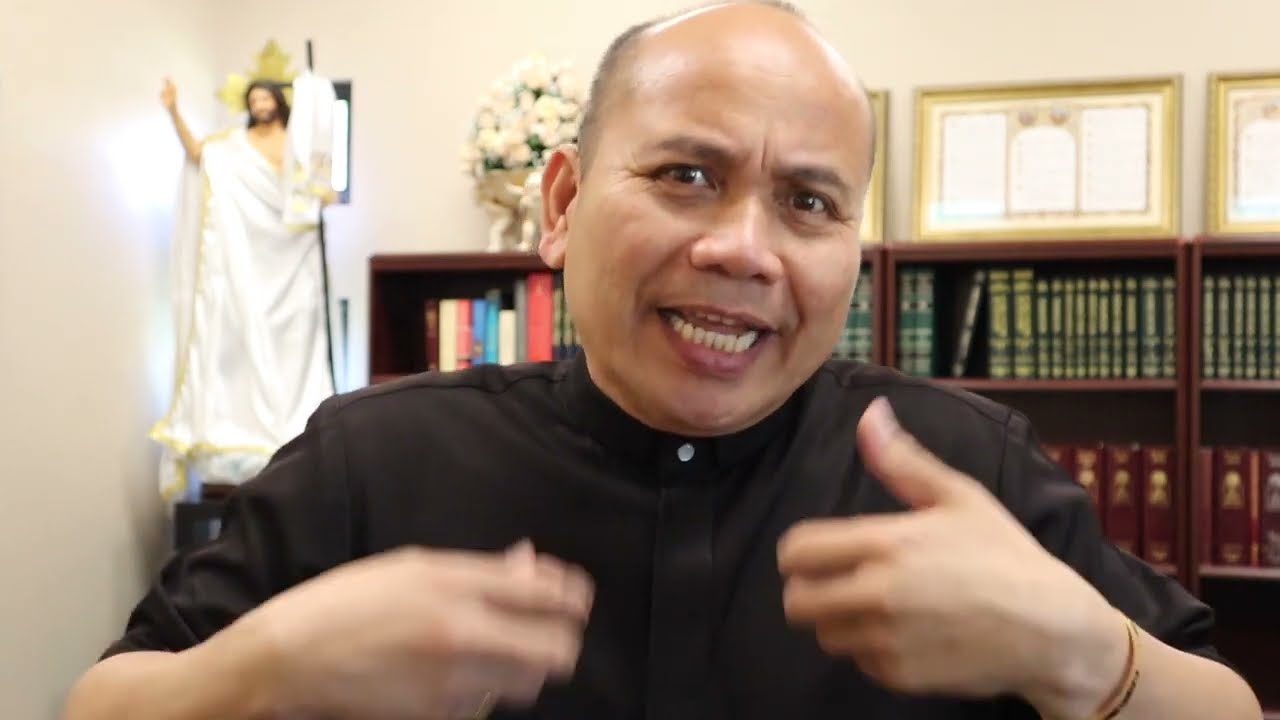In this image, a middle-aged man is seen from the chest up, appearing to be either sitting or standing. He is wearing a black short-sleeve shirt buttoned to his neck, with his arms bent at the elbows and raised to his chest, gesturing animatedly while speaking. His rounded face with olive skin and balding head, featuring closely cropped dark hair patches, is expressive as his mouth is open mid-speech. A rubber bracelet is visible on his left wrist. 

The background features a set of brown bookshelves filled with books, including encyclopedia sets with greenish and maroon-red covers, some plaques, and a potted plant on the left side. On top of the shelves, there are white flowers and golden frames. In the upper left-hand corner, a picture of Jesus dressed in a white garment holding a staff with an extended arm pointing upwards is noticeable. The walls of the room are a light beige color, contributing to the overall serene ambiance. The image has elements that suggest it might be a screenshot from a live streaming session, possibly on a platform like Facebook Live.